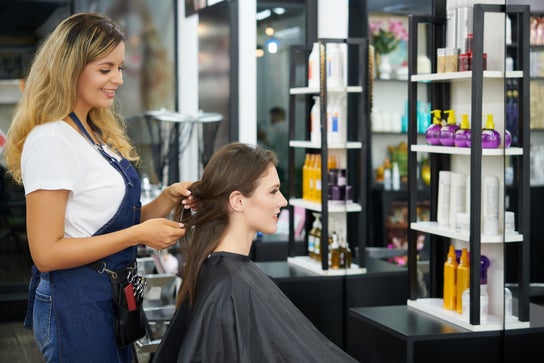In this professional photograph, likely intended for a magazine, two women are showcased in a vibrant salon setting. The focus is on a woman with straight brown hair and pale skin, who is seated and wearing a protective black stylist cape that obscures her clothes. Her hair is being styled by another woman standing behind her. The stylist has fluffier brown hair with dyed ends and is dressed in a white t-shirt paired with blue denim overalls. A leather tool belt, adorned with scissors and combs, is strapped around her waist. She smiles as she works on her client's hair.

The salon itself features multiple hair styling stations, each equipped with mirrors and shelves laden with an array of hair products. These products are mostly housed in plastic bottles of various colors, including orange, yellow, purple, and white. Some notable bottles are spray bottles with yellow tops, and others are shiny purple or white with labels. The background subtly fades from the forefront, enhancing the focus on the two women while still showcasing the busy, well-stocked environment of the salon.